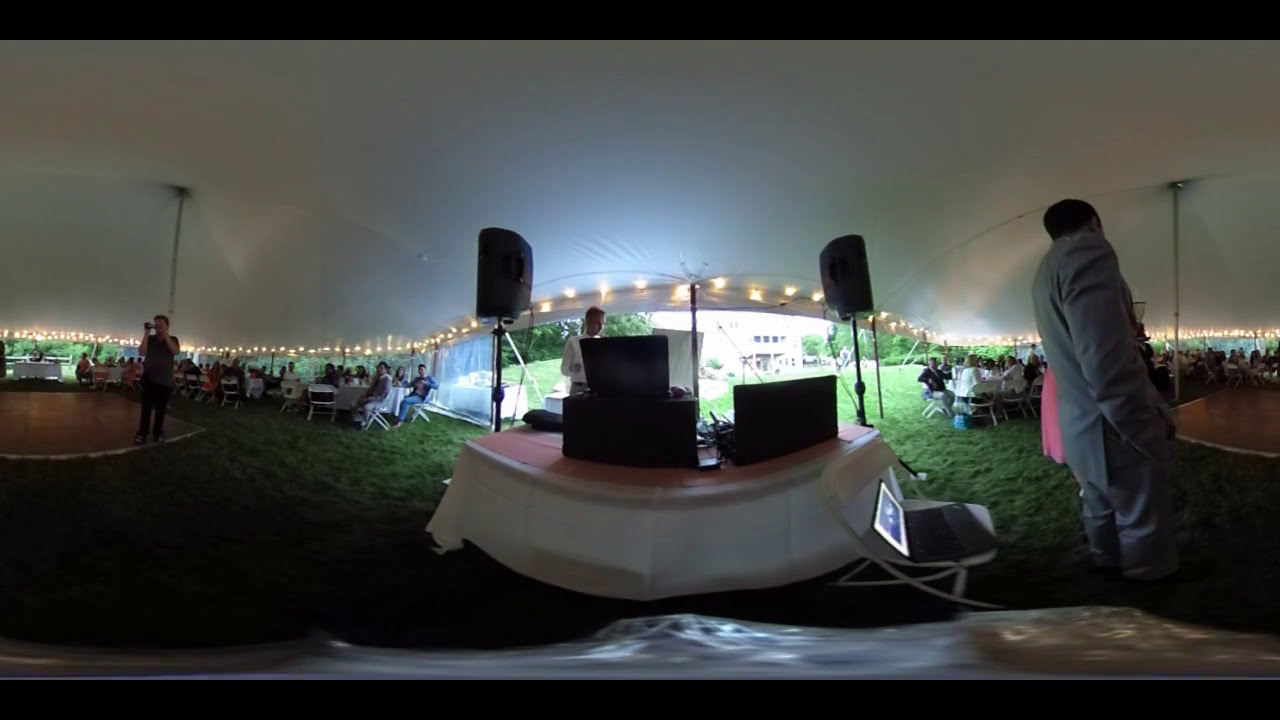Under the white-tinted canopy of a celebration, likely a wedding, a fisheye lens captures the scene, distorting the surroundings into a unique perspective. Central to the image is a table adorned with an orange tablecloth and partially covered by a white sheet that drapes to the ground. On the table, black boxes resembling speakers are stacked, presumably part of a sound system setup. To the right of the table, a white chair holds an open black laptop, its screen displaying a white background with a blue square. 

Further right, a man in a gray suit with dark hair stands facing a crowd, partially visible with his back turned leftward. The canopy's yellow string lights illuminate the scene, contributing to the festive ambiance. White chairs and tablecloth-covered tables seat guests on both sides of the canopy, with some attendees standing. 

To the far left, a round stage with a brown base hosts a man holding a camcorder, capturing the event. Outside the canopy's front entrance lies bright green grass, and a building with reflective black spots refracts light back into the canopy, enhancing the brightness inside. This carefully arranged reception scene provides a vibrant, celebratory atmosphere for an outdoor event under the expansive, softly lit canopy.